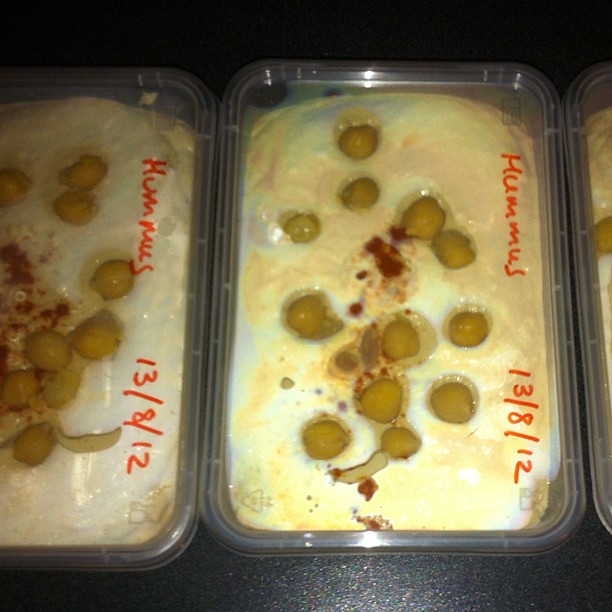The image is a color photograph likely taken in a deli or Middle Eastern food store, depicting at least three rectangular plastic containers filled with light brown hummus. The containers, which are disposable and made from clear, rigid plastic, feature lids that fit snugly without doming. The background is black, and bright lighting accentuates the scene despite the overall dark quality of the photograph.

Each container is labeled in red marker with the word "hummus" and the date "13-8-12," suggesting they were prepared on August 13, 2012. The hummus is garnished with whole green olives spaced across the surface, and there are scattered chickpeas and possible paprika or another reddish spice adding color and texture. The lids are clear, allowing a view of the contents, and sit indented rather than domed. The focus is on two prominently displayed containers, with a partial view of a third on the left side of the image.